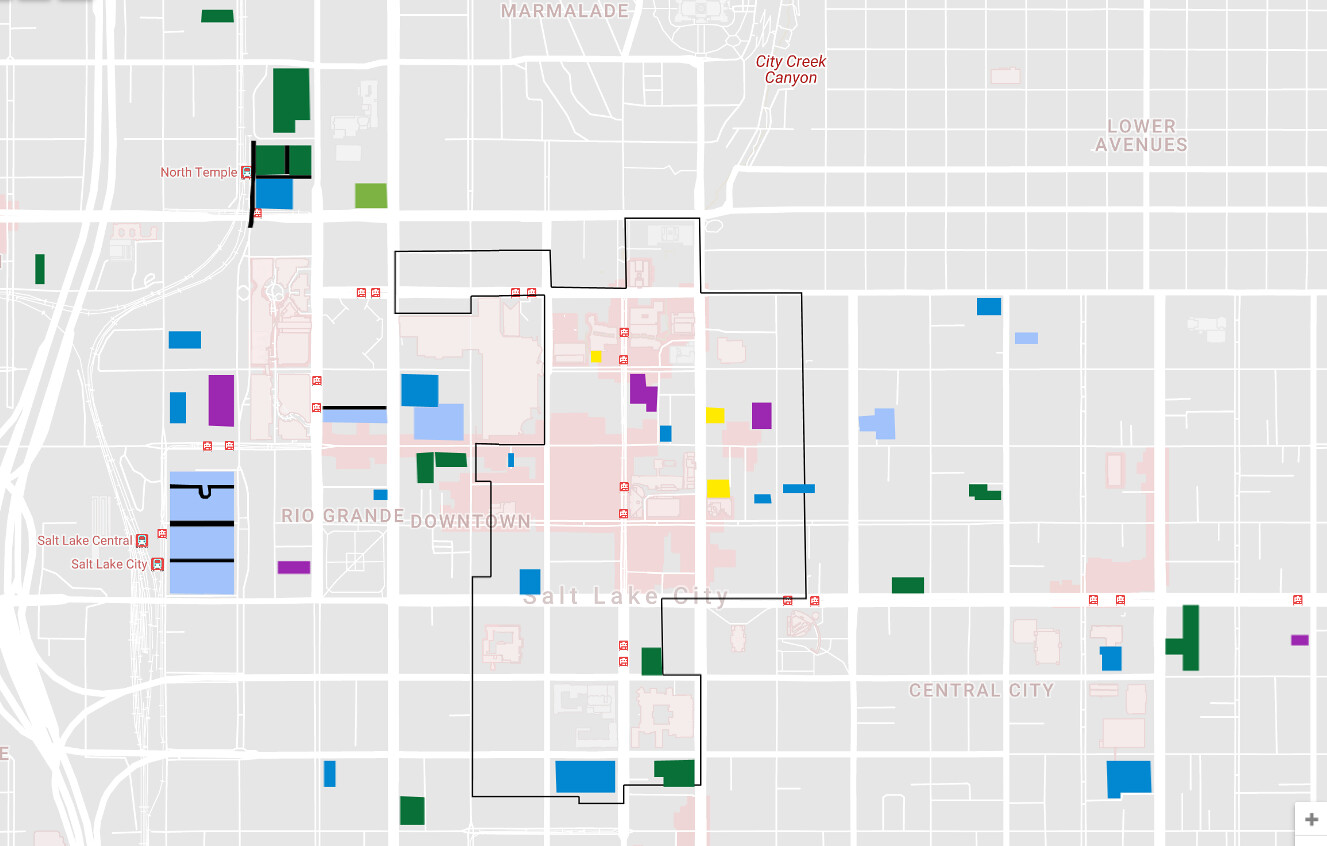This detailed map highlights an area of Salt Lake City with a minimalist design featuring gray and white backgrounds that emphasize the urban layout. City blocks and streets are clearly visible, creating a straightforward visual guide. Prominently labeled areas include "Lower Avenues" in the upper right corner, "Rio Grande Downtown" in the central portion, and "North Temple" toward the top left. Additionally, the "Marmalade" neighborhood is denoted at the top of the map. "Salt Lake City" is boldly displayed near the bottom center, affirming the map's focus. Unlike traditional maps, this one lacks a key and uses blocks of blue and green without explanation. Symbols of buses are visible on the left side, indicating routes to central locations like Salt Lake City and Salt Lake Central.